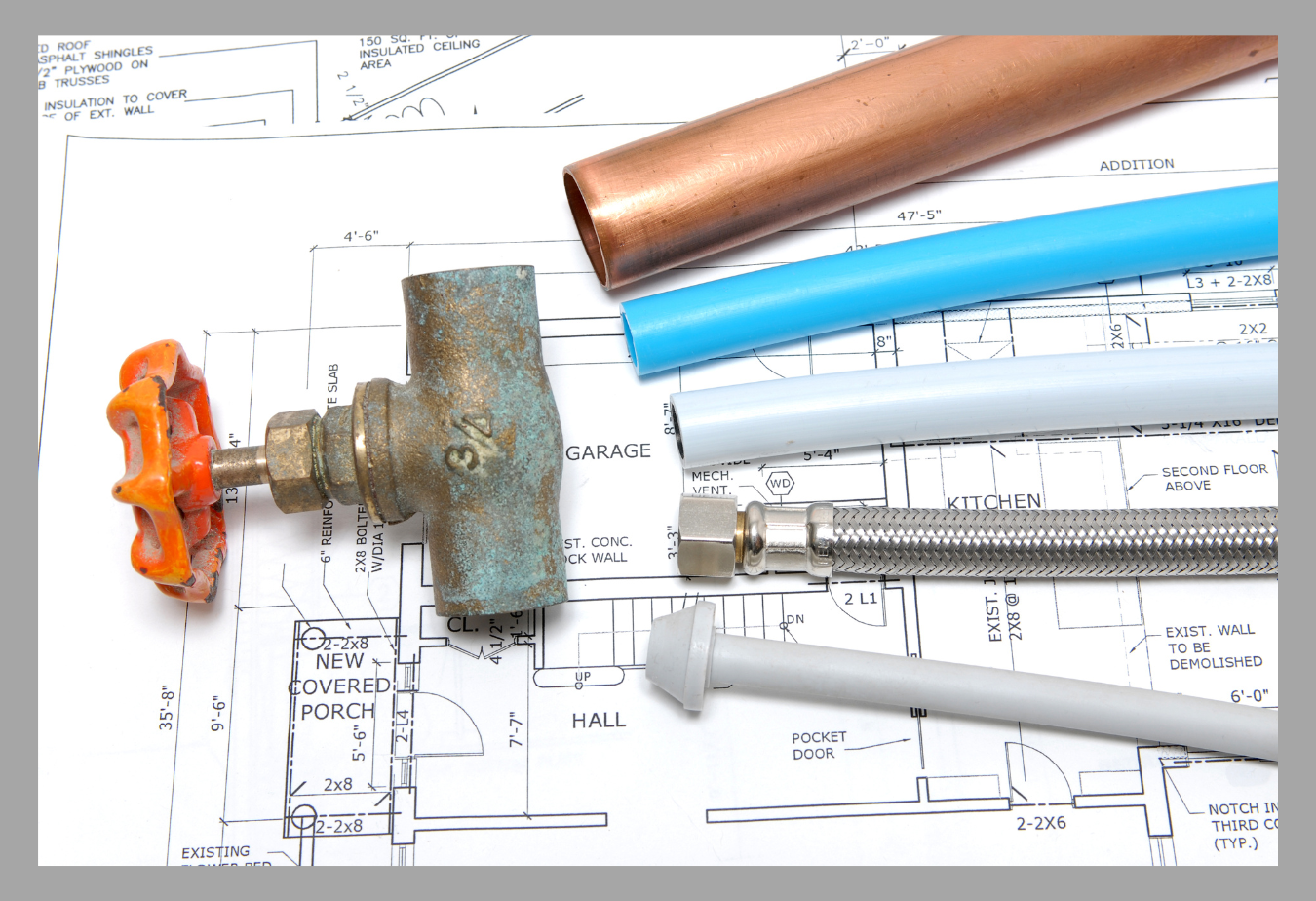This rectangular image, roughly six inches wide and three inches high, is framed by a thin, gray border about a quarter of an inch thick. Within this frame lies a white piece of paper featuring intricate blueprints in shades of black and gray. The blueprints detail various parts of a house, labeled with terms such as "new covered porch," "garage," "hall," "kitchen," and "pocket doors."

On the left side of the image, an oxidized, weathered three-quarter-inch valve with an orange twist handle is prominently placed. This valve, attached to a piece of copper piping that has started to turn greenish-blue due to oxidation, forms a T-shape. The copper pipe, etched with "3/4" indicating its size, is surrounded by various types of pipes and tubes that extend towards the right, partially disappearing off-screen. These include, from top to bottom, a bronze or copper tube, a blue plastic tube, a white PVC pipe, a silver braided cord tube, and finally, a thinner white plastic tube. All these elements rest atop the detailed blueprints, providing a technical and industrial contrast to the schematic background.